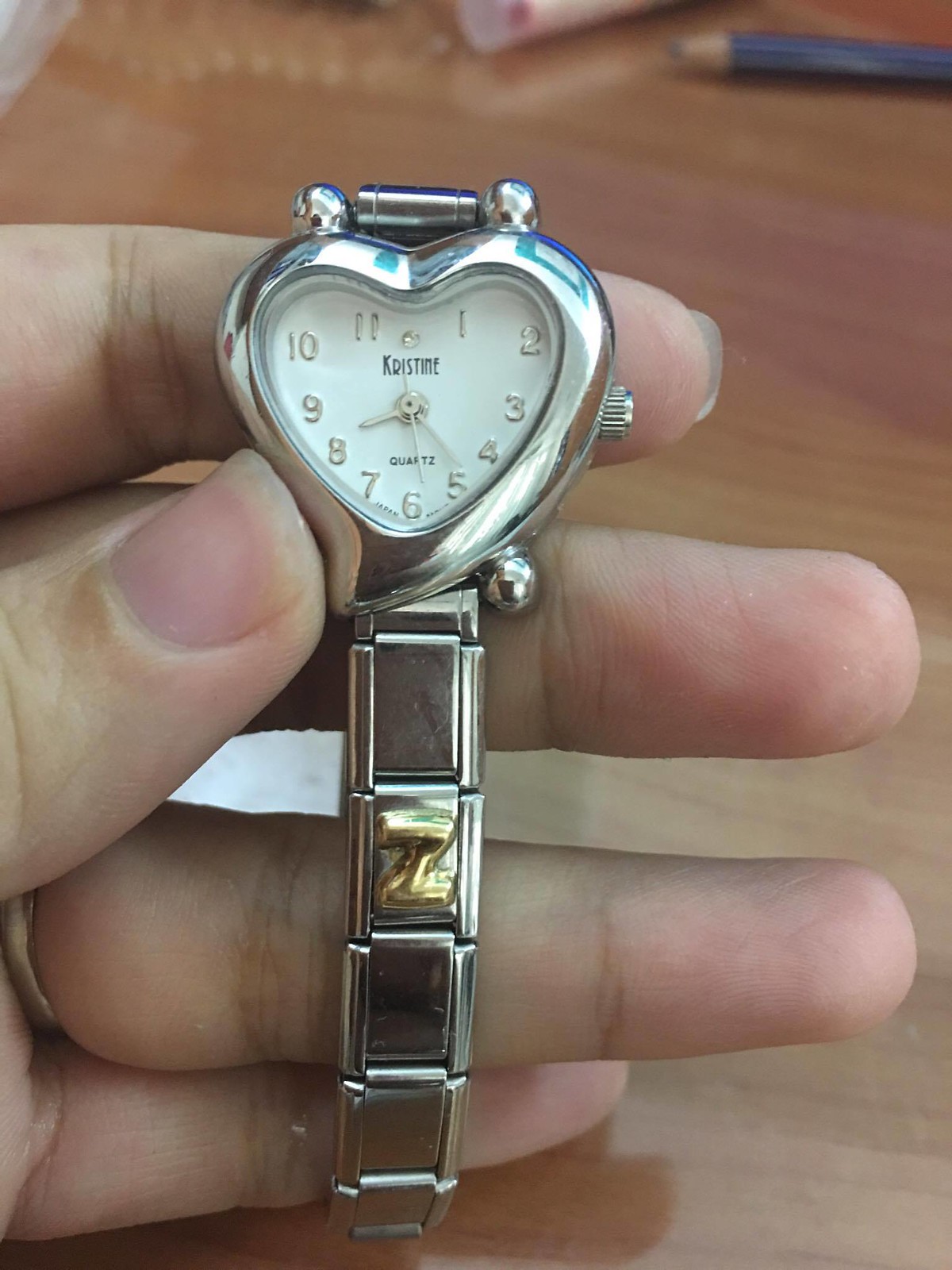In a detailed close-up photograph, a hand with light skin and long fingernails, possibly female, holds a heart-shaped wristwatch. The hand is positioned with the thumb pressed against the edge of the watch while the band drapes elegantly around the back of the fingers. The watch features a silver frame and a white face with the word "Christine" printed prominently in black at the center, and "quartz" inscribed below. The watch face is marked with a single dot at the 12 o'clock position, while the other hours are labeled 1 through 11 in metallic silver. The heart-shaped case swooshes downward to the left at the bottom, creating an asymmetrical design. The watch also boasts silver hour, minute, and second hands. The strap is composed of small, tile-like silver sections, with a distinctive gold 'Z' embellishing one of the segments. The background shows a slightly blurred wooden desk or surface with a pencil and other indistinct objects, emphasizing the sharpness of the watch and hand in the foreground.